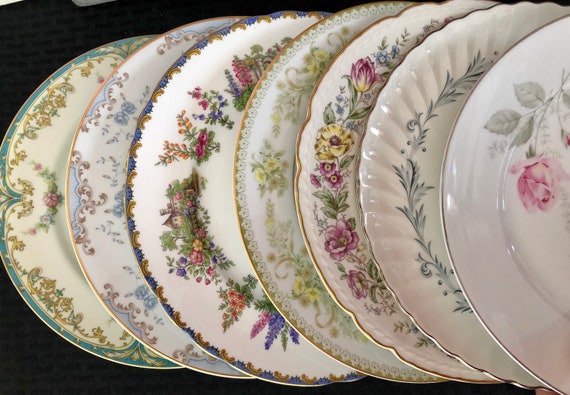This is a horizontal rectangular image showcasing a series of fine china plates, each standing on their edge in a staggered formation, likely supported by a holder behind them. The black background provides excellent contrast, making the various designs and colors of the plates stand out. There are seven plates visible in the picture, with only the edge of each one visible until the front plate, which is partially cut off by the image's frame.

The first plate in the front is plain white, adorned with a red flower and green leaves. The second plate, which features a scalloped edge, has grooves and displays gray or green leaves at its base. The third plate is fluted with a design that includes yellow and pink flowers and green foliage, accented by a gold rim edge. The subsequent plates also have floral designs and various edge details, with some having gold or silver rims, all in different shades of white ceramic.